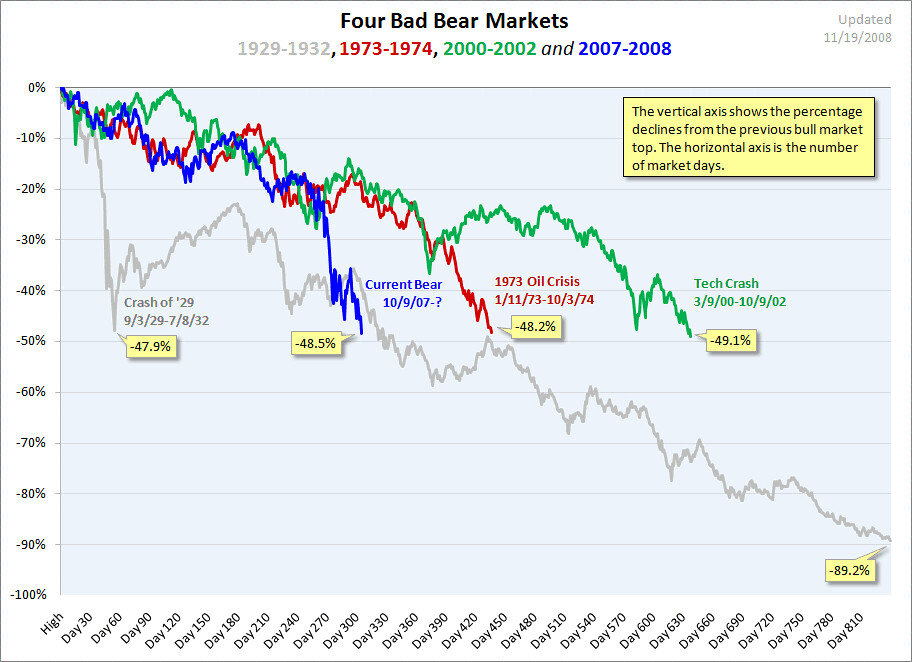The image portrays a detailed chart with a thin black border, titled "Four Bad Bear Markets" in prominent dark black text at the top center. This chart color-codes the four bear markets: 1929-1932 in gray, 1973-1974 in red, 2000-2002 in green, and 2007-2008 in blue. Located in the upper right corner is a yellow box with black text and a black border, indicating that the data was updated on 11-19-2008.

The vertical axis of the chart illustrates the percentage declines from the previous bull market top, ranging from -100% to 0% in increments of 10%. The horizontal axis represents the number of market days, starting from 'high', progressing in increments of 30 days up to 810 days.

Each market period is mapped out with statistics on the decline percentages: the Crash of 1929 is noted, as well as the declines from the 1973 oil crisis, the 2000 tech crash, and the figures for the 2007-2008 bear market. The chart provides a comprehensive overview of how each bear market unfolded over time.